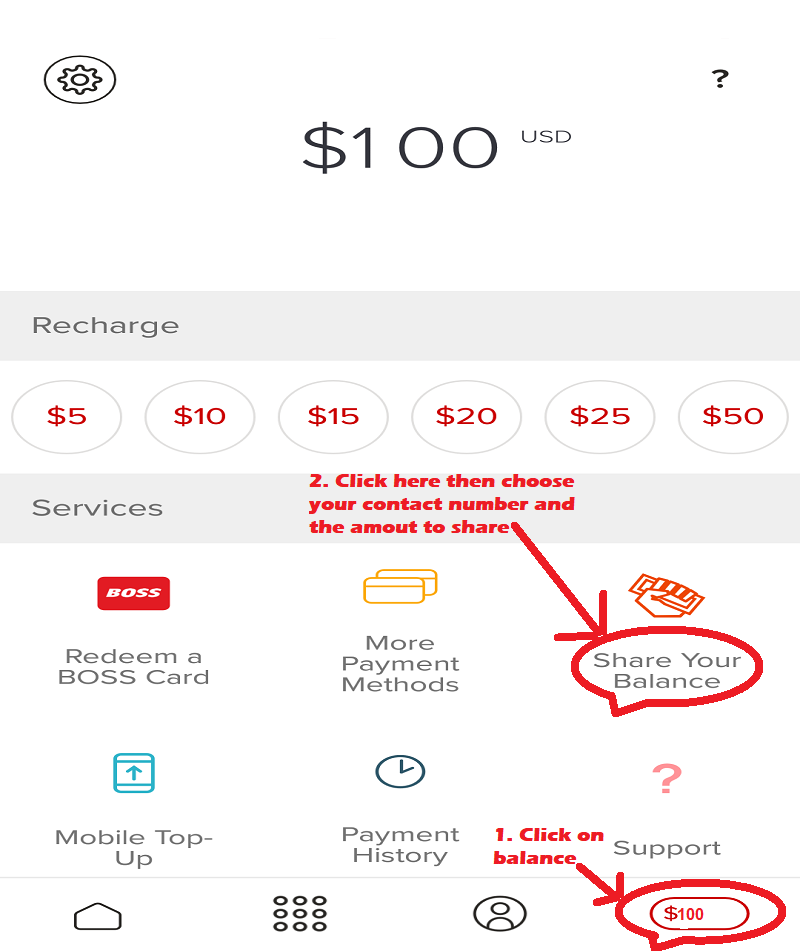The image features a white background with several components arranged meticulously. 

In the top left corner, a white circle bordered by black encloses a black settings icon. On the opposite side, in the top right corner, there is a black question mark.

Centrally placed at the top of the image, the text reads "$100 USD" in bold black font, with the dollar symbol situated to the left of the number and "USD" in smaller text to its right.

Below this, three horizontal rectangular boxes are aligned. The first and third boxes are light gray, labeled "Recharge" and "Services" respectively, both in gray text. Sandwiched between them, the middle box is white and contains six circular buttons outlined in light gray. These buttons feature monetary values in order: "$5" in red text, followed by "$10", "$15", "$20", "$25", and "$50" in black text.

Beneath the "$15" and "$20" buttons, in the third light gray box, red text says "2DOT. Click here, then choose your contact number and the amount to share." Adjacent to this text, a red arrow points diagonally to the bottom right, leading towards a red circle embellished with light gray text inside stating "Share Your Balance."

To the left side of the image are four separate texts aligned vertically: "Redeem a Boss Card," "More payment methods," "Mobile Top Up," and "Payment History."

Further to the right, additional red text marked "1DOT Click on Balance" is observed, associated with a smaller red arrow also pointing towards the bottom right. This arrow directs attention to another red circle containing a white oval outlined in red, which displays the amount "$100" with the dollar sign preceding the number inside.